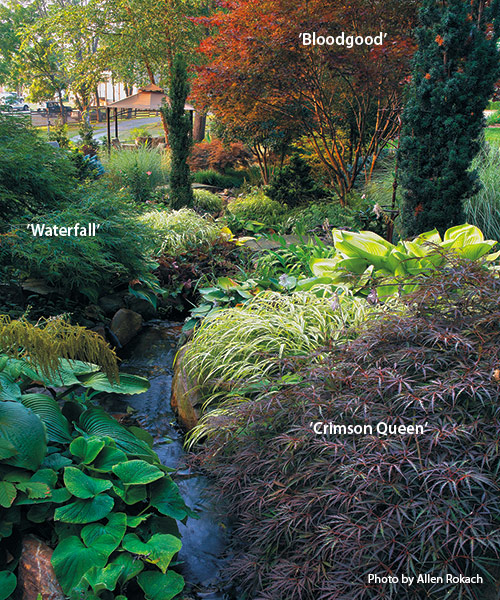The image depicts a dense and diverse garden park, rich with various trees and plants, creating a realistic and vibrant scene. In the foreground, a purplish-green plant is labeled "Crimson Queen" in white text. To the left, amidst the lush greenery, a plant named "Waterfall" is identified, featuring bright green, lily pad-like leaves. Further back in the scene, a small tree with burnt orange and red foliage is labeled "Bloodgood." Additional elements in the scene include green shrubs, rocks, trees, and what appears to be a patio or pathway that weaves through the dense plant life. The photograph features an array of colors—green, purple, blue, brown, red, and orange—capturing the diverse flora. The bottom of the image bears the text "Photo by Alan Rickson."